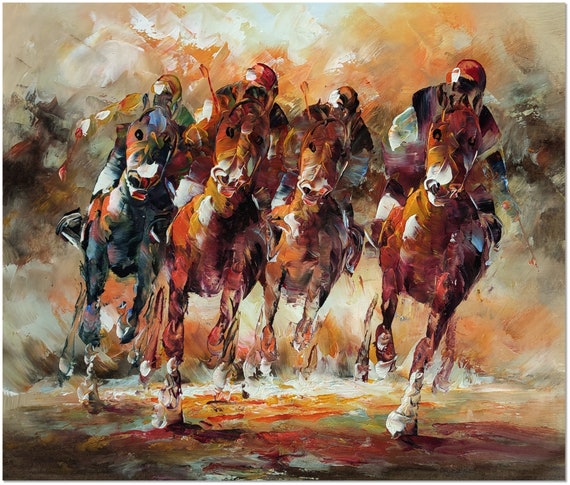This abstract watercolor painting vividly captures a dynamic scene of four jockeys riding racehorses, evocative of a prestigious event such as the Kentucky Derby. The horses, with muted tones of dark brown, gray, and black, gallop in a slight rightward slant, implying a vigorous turn or bend in their race. The jockeys, hunched over in their saddles, sport helmets in shades of red and orange, and at least three of them grip small whips in their hands. The background is a swirling blend of abstract smudges in orange, white, green, gray, and black, rendering the scene so dreamlike that the horses appear to be charging through puddles of paint rather than solid ground. Despite the abstraction, the horses' forms are discernible, embodying a striking beauty amidst the artistic chaos.